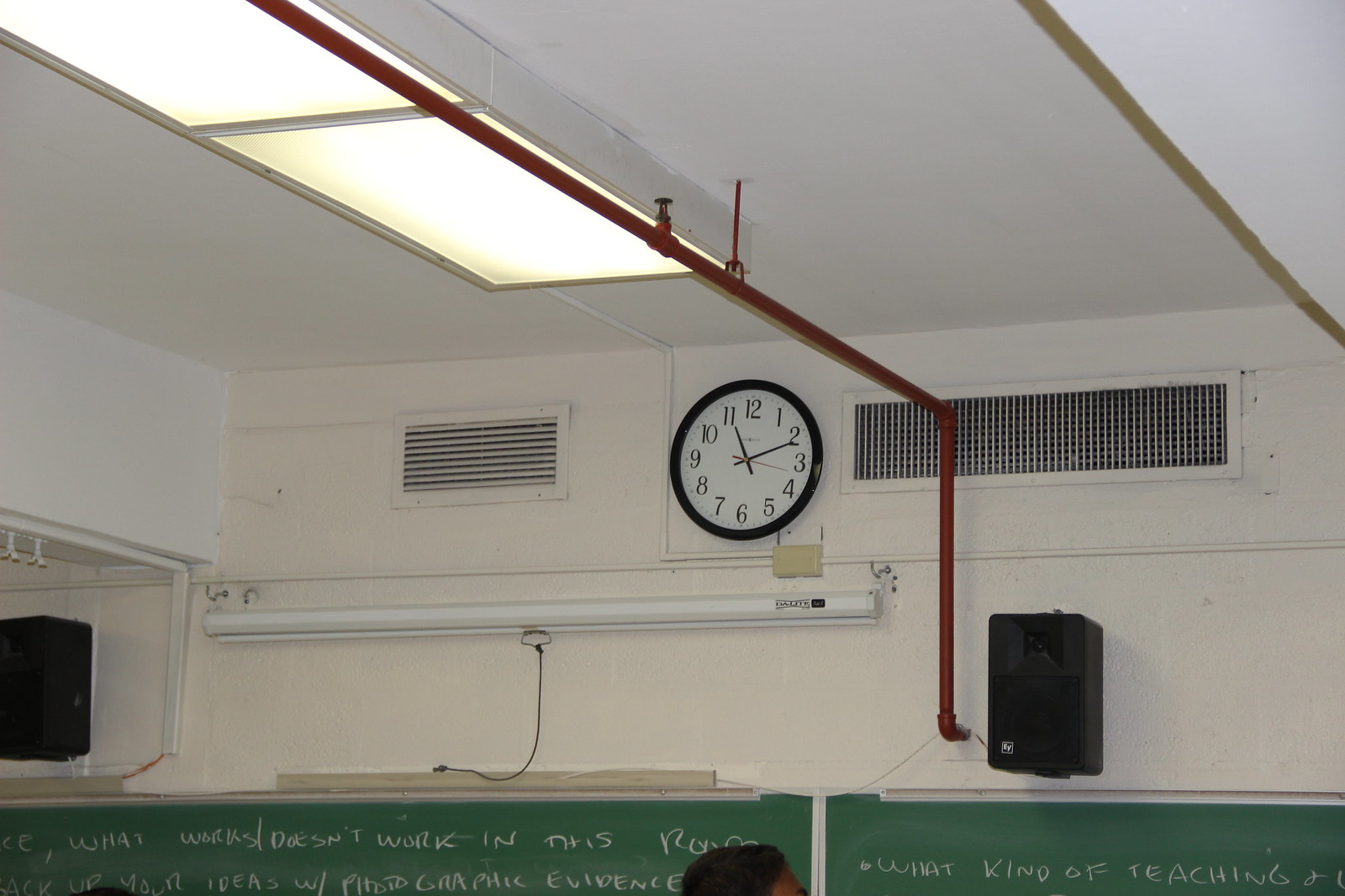The photograph appears to have been taken in a college classroom setting, focusing on the ceiling and the upper portion of the wall. At the bottom of the image, the top of an older male's head is visible, likely that of a professor or teacher. Two green chalkboards dominate the lower half of the frame, covered in handwritten English text relating to the concept of "What doesn't work in this?" followed by "Ideas with photographic evidence," although the remainder of the text is cut off, making it partially unreadable.

The wall above the chalkboards is painted white, punctuated by two mounted speakers and a roll-down projector screen. As the eye moves upward, you notice wall vents and a prominent red pipe that starts at one of the speakers, running up along the ceiling. The ceiling itself is outfitted with fluorescent yellow lights. Near the top of the image, a clock is prominently displayed, showing the time at approximately 11:10 or 11:11. The arrangement and elements suggest a well-equipped, modern educational environment.